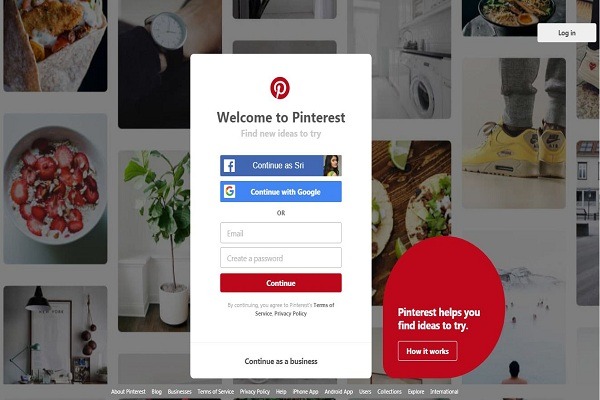In the image, we observe a welcome page for Pinterest. The prominent text reads, "Welcome to Pinterest. Find new ideas to try." The page offers several options to proceed: "Continue as Siri," "Continue with Google," or by manually entering an email and creating a password in the provided fields. The "Continue" button is highlighted in red with white text. Below this, there is a disclaimer stating, "By continuing, you agree to Pinterest's Terms of Service and Privacy Policy." Additionally, there's an option to "Continue as a business."

The footer of the page includes various navigational links such as "How it works," "About Pinterest," "Blog," "Business," "Terms of Service," "Privacy Policy," "Help," "Phone app," "Android app," "iPhone app," and "Explore." The page is visually accented with colors like blue, red, and white.

In the background, there are miscellaneous items including food, a clock, plants, sneakers, and a laundry room, which add a vibrant and everyday life ambiance to the scene.